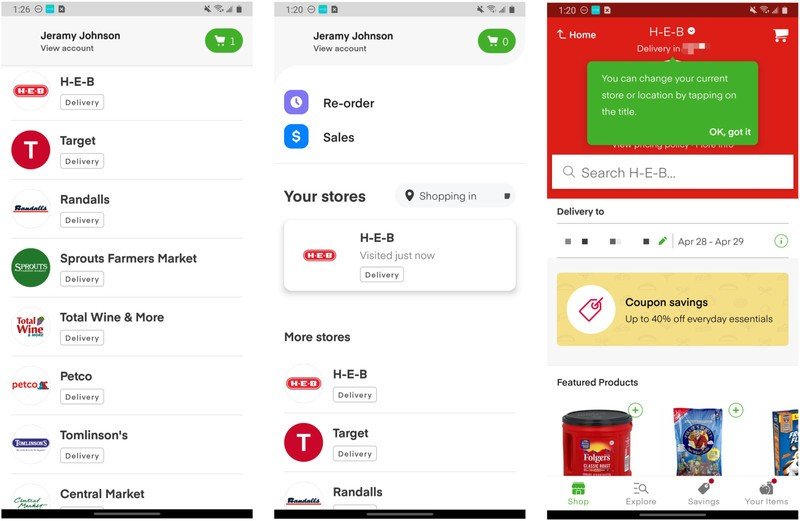The image comprises three sequential screenshots from a mobile device.

**Screenshot 1:** The first screenshot shows a mobile interface with 126 notifications turned off, Wi-Fi enabled, and full battery life. At the top, the user's view is attributed to Jeremy Johnson, with a green button featuring a cart icon displaying the number one. Below, it lists various delivery stores including HEB Delivery, Target Delivery, Randall's Delivery, Sprouts Farmer's Market Delivery, Total Wine & More Delivery, Petco Delivery, Tomilson's Delivery, and Central Market.

**Screenshot 2:** In the center screenshot, Jeremy Johnson is featured again, with the current time displayed as 1:20. A blue button labeled "Reorder" with a clock icon and a dark blue button labeled "Sales" with a money symbol are visible. The section "Your Stores" shows HEB highlighted and marked as "Visited Just Now."

**Screenshot 3:** The final screenshot includes a red banner at the top with the time still at 1:20. It displays a home icon with a back arrow next to HEB, indicating the selected store. A green pop-up advises that the current store or location can be changed by tapping on the title, accompanied by a confirmation button stating "Okay, got it."